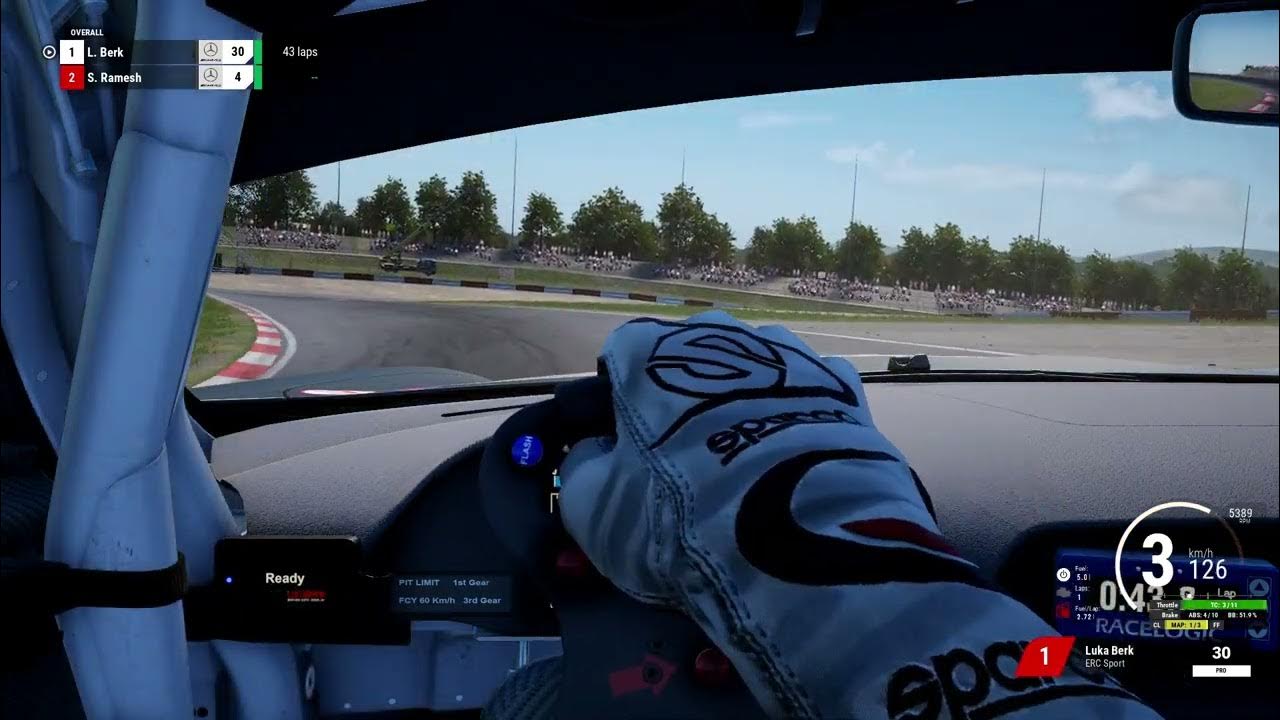The image depicts a detailed scene from an auto-racing video game. In the top left corner, L. Burke, identified as the player, is highlighted, being sponsored by Mercedes. Displayed prominently is that he is currently on lap 30 out of 43. In second place, marked in red, S. Ramach, also sponsored by Mercedes, is noted, although his lap count is not visible.

The interface includes various indicators and instructions: one area says "ready" and another indicates "pit limit first gear" at "CY60 KMH third gear." The speed is shown as 126 kilometers per hour, represented within a white semi-circle. Below this, a series of colored bars—green, black, and yellow—contain unreadable text. The leaderboard highlights L. Burke in first place under ERC Sport, with '30' next to his name. A white bar labeled 'PRO' in black text implies a professional level or ranking.

The in-game view features the dashboard of the racing car, with the player’s hand, adorned in red and white racing gloves, gripping the steering wheel. The car's interior displays white roll bars and a rear-view mirror mounted on the ceiling. The exterior view captures the race track, flanked by red and white barriers, and spectators in the stands are visible in the distance. The scene conveys the intensity and realism of the racing simulation.